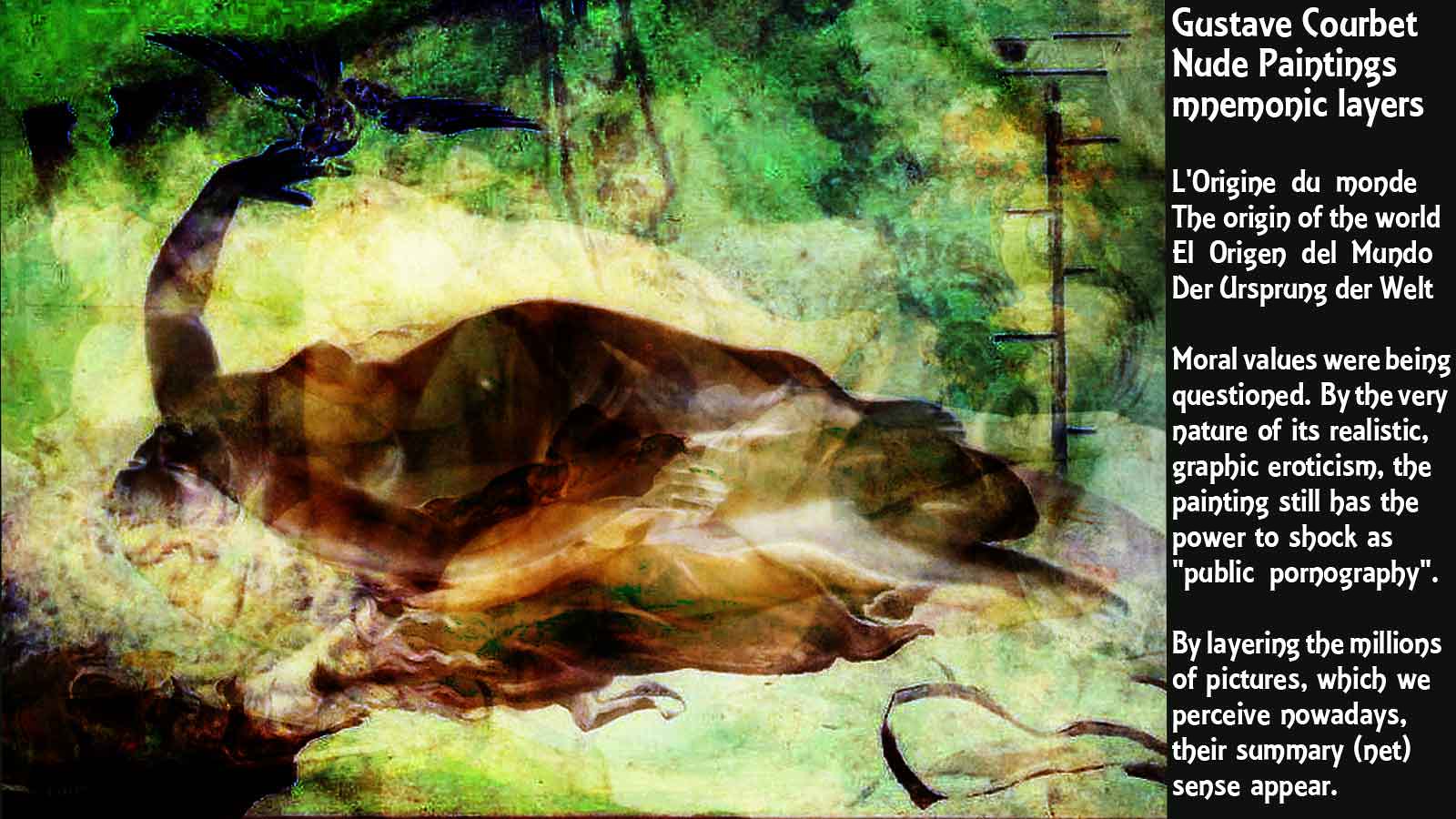The image features a visually complex and abstract scene, combining dark and vibrant colors. On the left side, two images are layered on top of each other, creating a composite visual that includes a nude figure. The figure is reclining and has a dark brown body with hints of purple hues and yellow hair. One of her raised hands, cast in purple, holds a black bird, while the background is interspersed with green vegetation, grass, and possibly trees and bushes, though the exact details are blurred and hard to discern.

On the right side of the image, set against a black background, is white text that reads: "Gustave Courbet, Nude Paintings, Mnemonic Layers, Lorraine de Monique, The Origin of the World, El Origen del Mundo, Der Ursprung, Del Vuelto." Below this, the text comments on the provocative nature of the painting: "Moral values were being questioned by the very nature of its realistic graphic eroticism. The painting still has the power to shock as public pornography. By layering the millions of pictures which we perceive nowadays, there is some re-knit sense of pure."